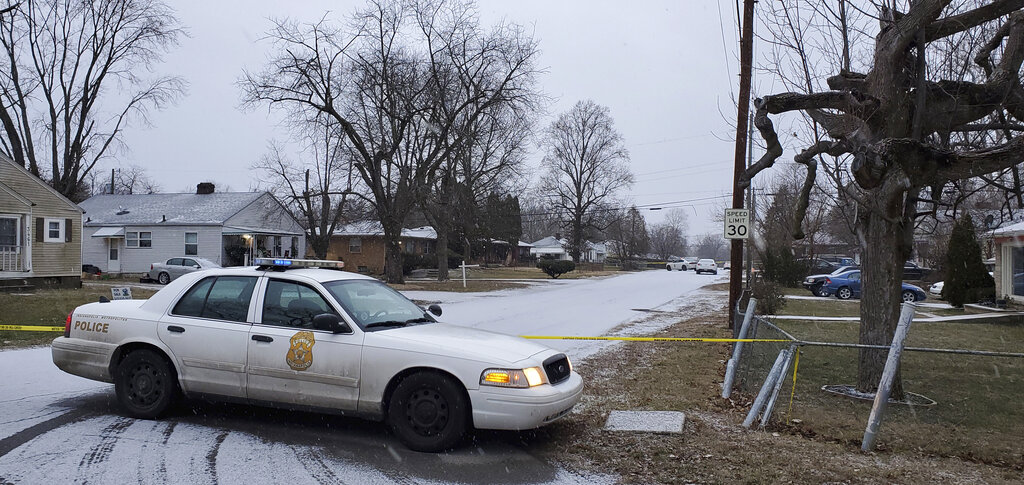The photograph depicts a white police car with its headlights on, parked at an awkward angle, possibly executing a U-turn. The vehicle is identifiable by the rooftop light bar, although no officers are visible inside. The setting is a residential neighborhood with small brick houses on either side and cars parked in their driveways. The area is cordoned off by yellow police tape, suggesting a recent incident. A 30 mph speed limit sign is mounted on a brown wooden pole next to a twisted, leafless tree. Overhead, power lines stretch across a dull gray sky, which has a faint hint of blue. The street appears to be dusted with snow, although curiously, the grass remains mostly clear. A slightly bent chain link fence is also visible, adding to the sense of urgency and disruption in this ordinarily quiet setting.